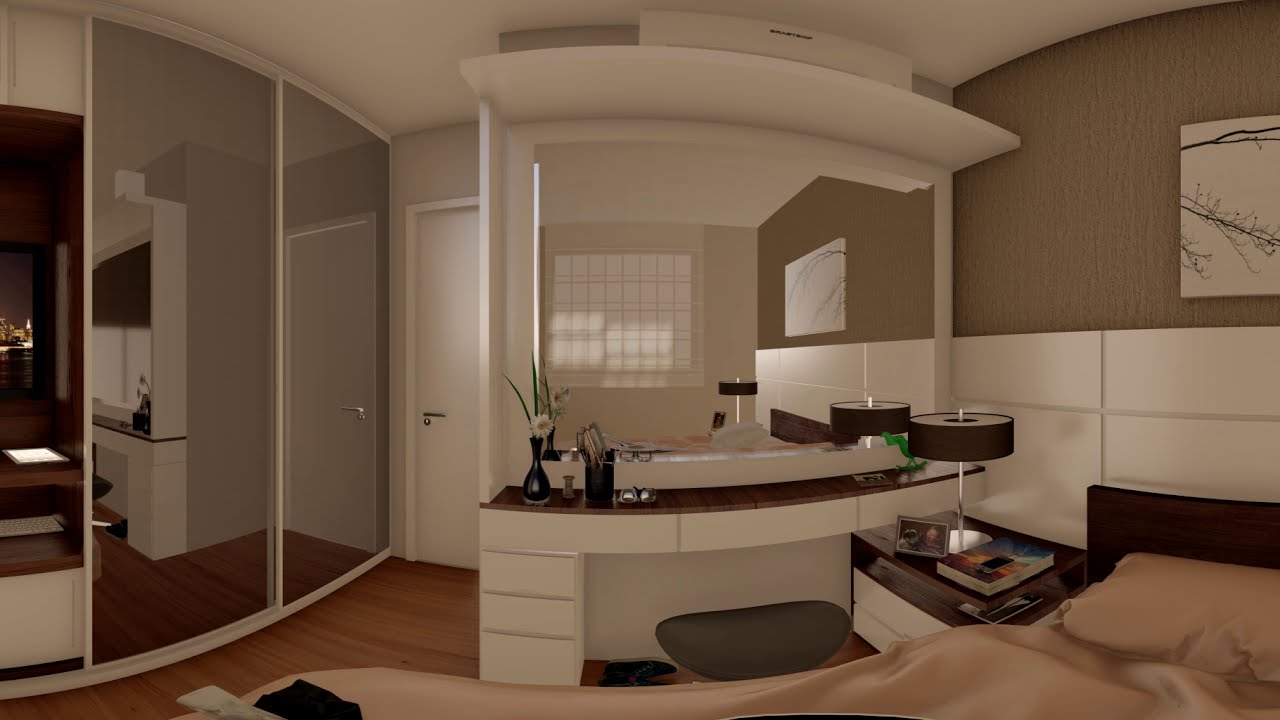The image depicts a digitally created, full-color visual of what appears to be a hotel room or master bedroom, captured from a slightly warped, fisheye perspective. The room features a bed adorned with a light tan blanket and pillow, accompanied by a dark brown headboard against a backdrop of a half-white tiled lower wall and a light brown upper wall. A white painting of a tree branch hangs just above the white panel. To the right of the bed, there is a dark brown nightstand with white drawers underneath and a silver lamp with a round brown lampshade on top. Adjacent to the nightstand is a white dressing table with a large mirror and a small stool. The vanity area includes a lamp, a book, a photograph, glasses, and a small flower arrangement. To the left of this setup, there is a white door with a handle typical of hotels, and mirrored sliding closet doors. The presence of a computer or laptop on a small side table completes this meticulously detailed and homely interior scene.